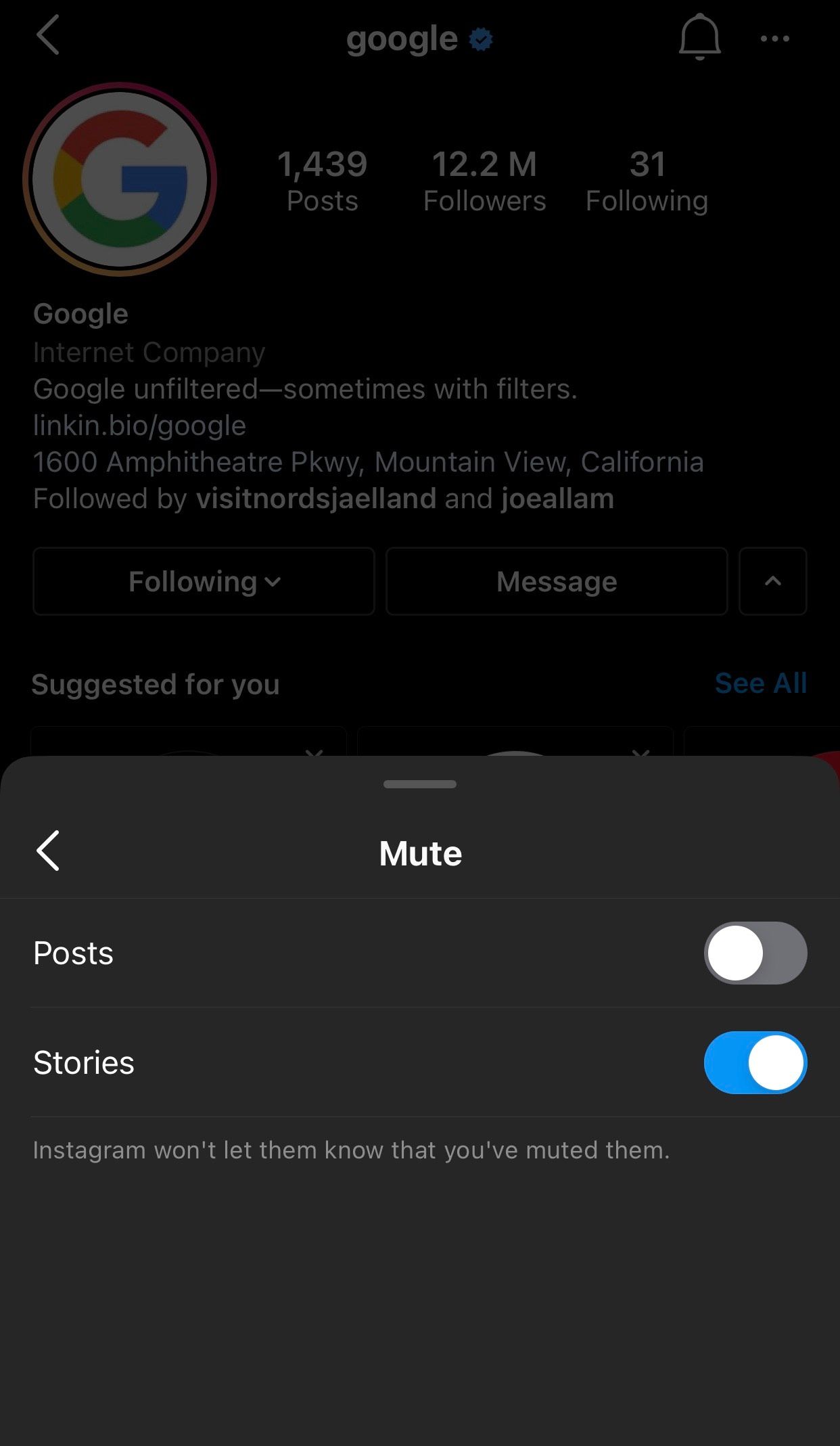This is a screenshot from a mobile device, featuring an overlay that gives the image a faded appearance. The outer edges of the phone are not visible, only the screen's content is shown. In the top left corner, there's a left-pointing arrow. Centered at the top is the word "Google" in lowercase text. To the right of "Google" is a blue circle with a check mark inside, followed by a bell icon and three vertical dots.

Near the top left of the screen, the iconic multicolored "G" for Google is displayed within a white circle that has a golden-reddish trim. Below this logo are labels for "Posts," "Followers," and "Following." Underneath, the word "Google" appears again with the subtitle "Internet company." The following line reads, "Google unfiltered sometimes with filters," and then "link in bio / Google." 

Further down the screen, the address "1600 Amphitheater Parkway, Mountain View, California" is listed. There is a call to action, "Visit," followed by information about "Nor dsj a ell and and Joe Alla." This is followed by the options "Following" with a drop-down arrow and "Message" with a drop-up arrow.

Under the section "Suggested for you," there is an option to "See all." At the bottom of the overlay, navigation options read "Muted" with a left arrow beside it, alongside toggles for "Post" (off) and "Stories" (on).